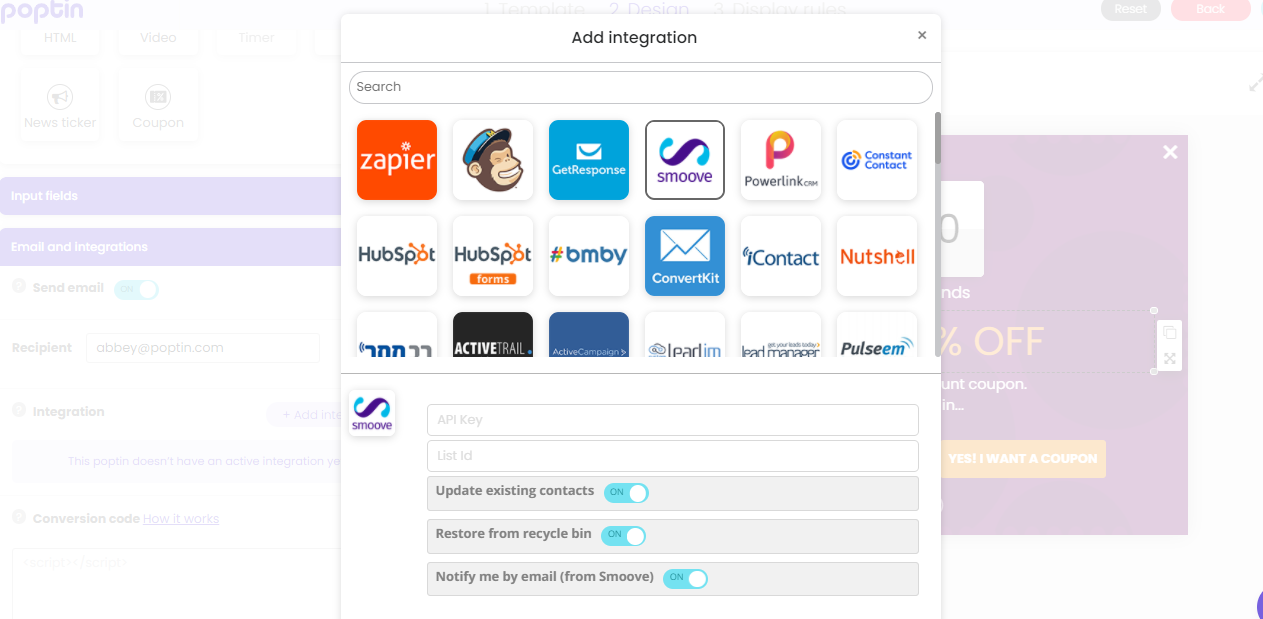The screenshot features a website interface prominently displaying the company's name, "popbin," in lowercase letters (p-o-p-b-i-n) on the left side. The background is slightly blurred, emphasizing the central focus: a white pop-up box. At the top of this box, the text "Add Integration" is conspicuously placed, followed by a search bar.

Beneath the search bar, a series of icons representing various contact management software services are displayed in a horizontal arrangement. From left to right, the visible icons include:

1. **Zapier**: Recognizable by its distinctive logo.
2. **MailChimp**: Depicted by the iconic cartoon head of a chimpanzee wearing a blue cap.
3. **GetResponse**: Represented by a blue square with the service name written in white.
4. **Smooth**: Shown as a white square with a stylized sideways "S" logo.

Additional services listed include Powerlink, Constant Contact, HubSpot, ConvertKit, and iContact among others. These icons collectively represent a variety of contact management tools available for integration within the popbin platform.